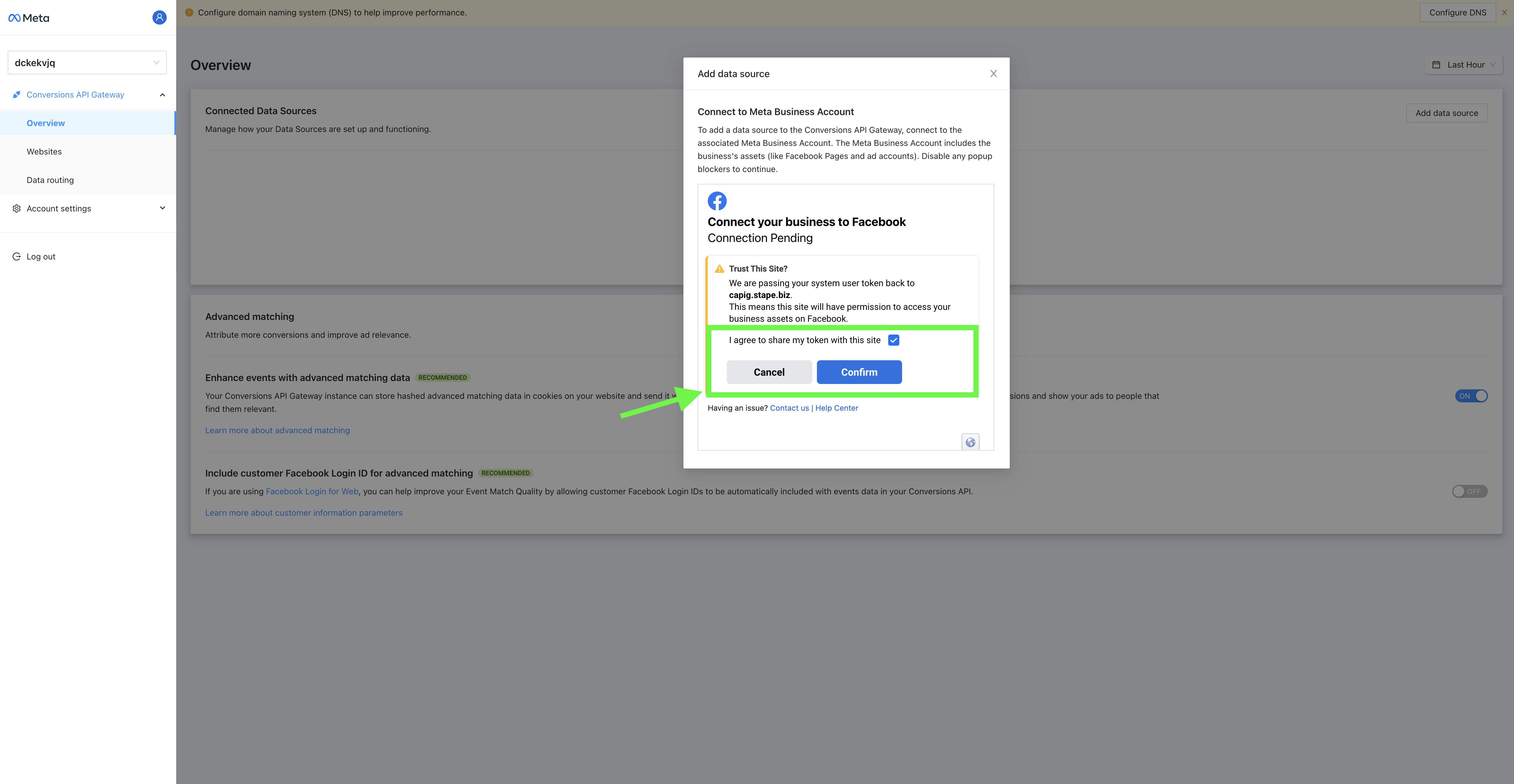This is a detailed caption for a screenshot of a web page interface, focusing on a specific section and various elements within it:

The screenshot captures a web page predominantly divided into two sections. On the left, set against a clean white background, is a vertical navigation column. At the top left of this column, there's a distinctive blue "Meta" logo accompanied by the word "meta" in black text. Adjacent to the logo is a blue generic profile picture icon.

Under the profile icon, there's a text box pre-filled with the lowercase text "dckekvjq." Directly below this is a blue hyperlink reading "Conversions API Gateway," followed by a menu of options. The "Overview" option is highlighted in pale blue with dark blue text, indicating it is currently selected. Below the "Overview" are the options "Websites" and "Data Routing," both in gray text. Further down the menu, under a different section labeled with a cog icon as "Account Settings," there's an additional item marked "Log Out" with a 'G' logo next to it.

The right section of the page, which constitutes the main content area, displays a prominent pop-up with a white background titled "Add Data Source." The text below reads, "Connect to Meta Business Account. To add a data source to Conversions API Gateway, connect to the associated Meta Business Account. The Meta Business Account includes the business's assets like Facebook pages and ad accounts. Disable any pop-up blockers to continue."

An illustrative Facebook logo is then followed by a status message stating, "Connect your business to Facebook. Connection pending." An overlay message further details, "Trust the site. We are passing your system user token back to CAPIG.stape.biz. This means the site will have permission to access your business assets on Facebook. I agree to share my token with the site." There is a checked blue checkbox indicating agreement to share the token.

At the bottom of this pop-up are two buttons: a gray "Cancel" button with black text and a blue "Confirm" button with white text. The remaining part of the web page in the background is significantly darkened, emphasizing the pop-up in the foreground.

This descriptive caption provides a thorough visual representation of the web page's layout and specific elements within the screenshot.